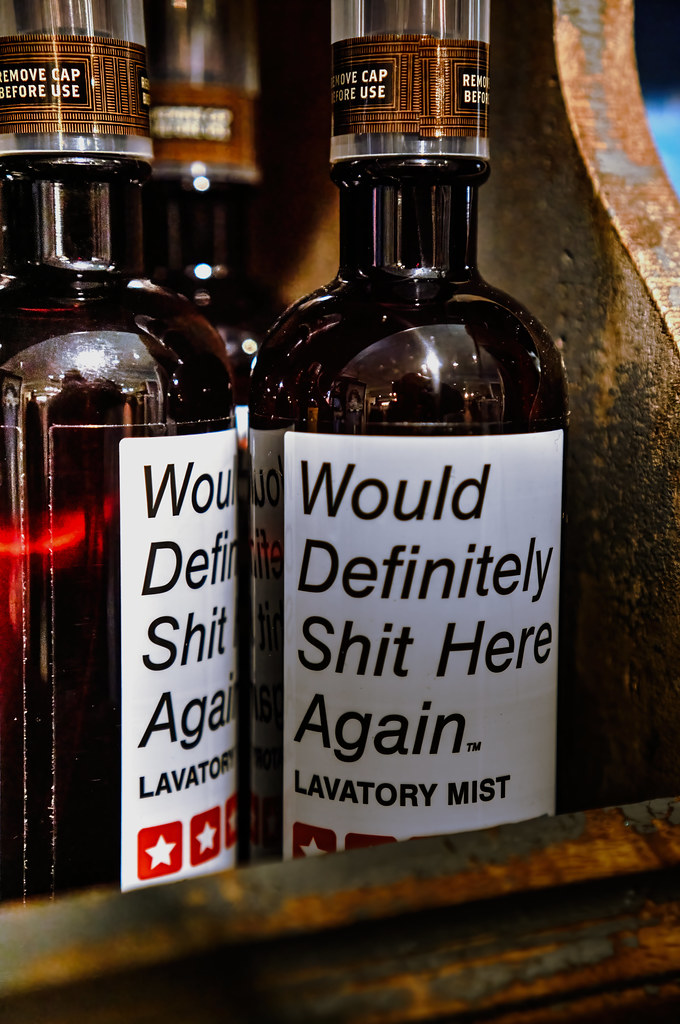The image captures three identical bottles of a product labeled as "Would Definitely Shit Here Again, TM Lavatory Mist." The bottles are brown and feature white labels with simple black lettering. Below the product name is a star rating section, with red star icons indicating user reviews, presumably a five-star rating based on visible red boxes with white stars. Two bottles are prominently positioned side by side, with one turned partially to the side making it harder to read the label, while a third bottle is situated in the background. The bottles are set within an old, worn, and rusty metal holding device that has a rich patina, giving it a vintage or weathered appearance. Each bottle has a clear cap marked with the instruction "Remove Cap Before Use." The overall setup suggests the product is a humorous bathroom air freshener.